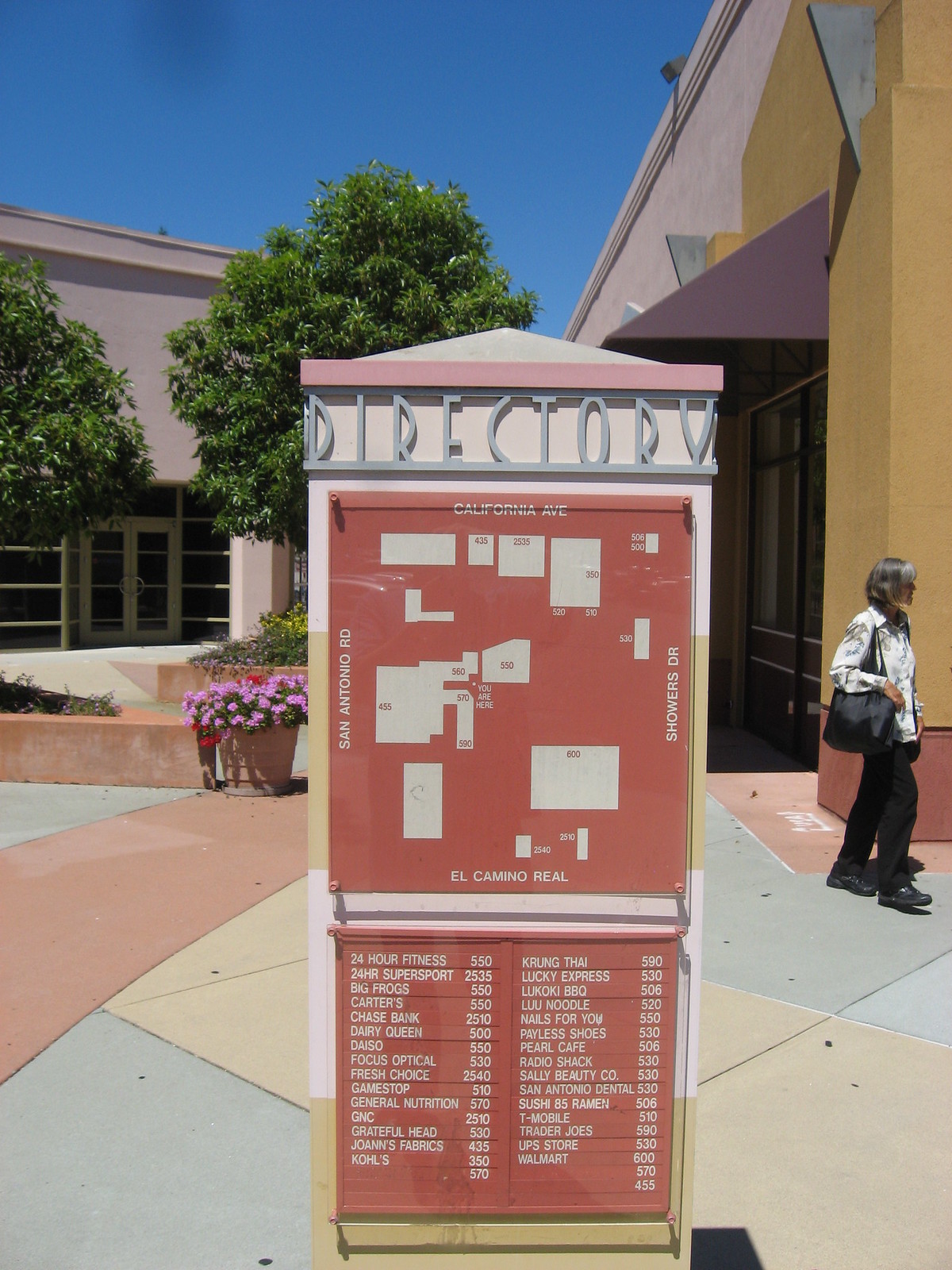This image captures an outdoor mall directory centrally located in what appears to be a warm climate, possibly in California, given the references to California Avenue, El Camino Real, San Antonio Road, and Showers Drive. The directory itself is brown with "Directory" written in green on a white peaked top. Below this title is a detailed map of the mall and the surrounding streets, with a list of stores categorized underneath. Visible store names include Chase Bank, Kohl's, Walmart, Trader Joe's, Dairy Queen, 24-Hour Fitness, Joann Fabrics, GameStop, T-Mobile, and many others.

Adjacent to the directory, on the right side of the composition, stands a clay planter filled with vibrant purple and red flowers. A line of clay bases, possibly housing small trees, can also be seen, hinting at the mall's aesthetic cohesion with earthy, sand-colored tones resembling architectural styles found in regions like Arizona.

In the foreground to the left stands a woman dressed in a white jacket and black pants, carrying a black bag over her right shoulder. The ground beneath her features a harmonious pattern of green, tan, and clay colors, echoing the building and planter designs. Triangular and square patterns embellish the concrete floor. The sky above is clear blue, and various trees frame the scene, enhancing the feeling of an open-air, sunlit environment.